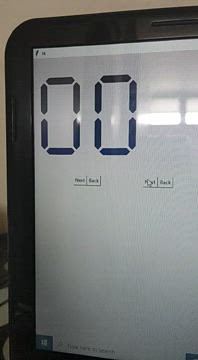The image depicts a black laptop or possibly another liquid crystal display device, set against a beige or brownish wall. On the screen, there are two digital zeros ("00") in black, likely representing a stopwatch or timer. Below these zeros are four buttons, two on the left side and two on the right, with labels such as "back" and "next." The screen has a thick black bezel around it. In the bottom left corner of the screen, there's a small gray square with a white Windows logo inside, adjacent to a white search bar with indecipherable text. The background of the screen is mostly off-white, and a white mouse arrow is visible over one of the elements. The top left of the screen also features a white bar, potentially indicating a Wi-Fi signal.